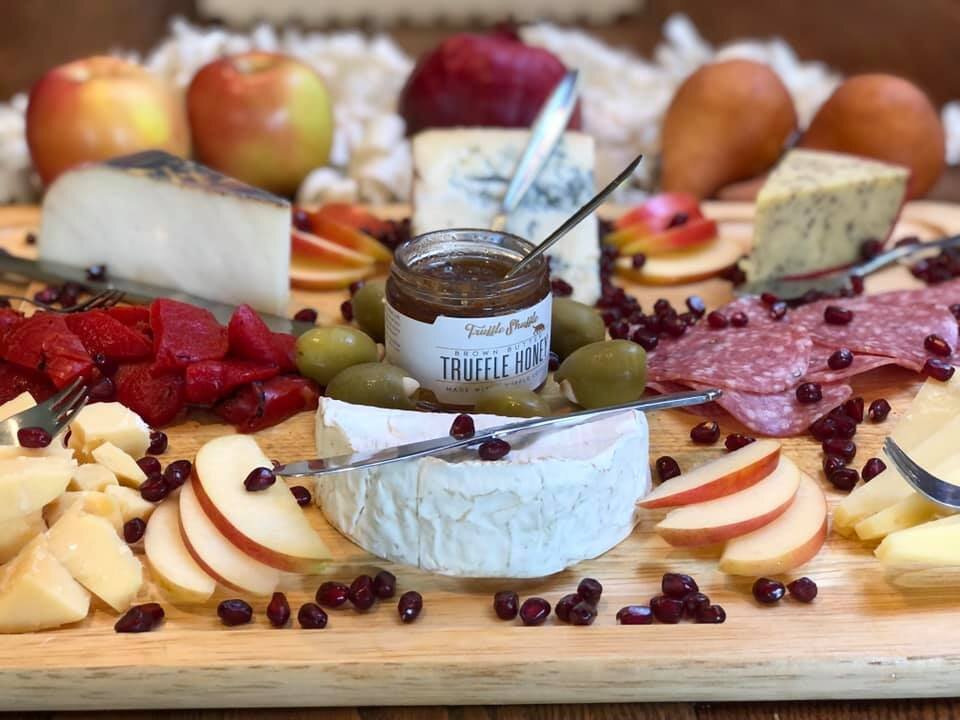The photograph depicts a charcuterie board, elegantly arranged on a light-colored wooden board that features a groove track along the edge. Central to the board is an open jar labeled "truffle honey," with a spoon inside. Surrounding the jar are a myriad of foods: In the foreground, there's a mix of sliced apples and pears, some neatly arranged while others are scattered, and some uncut apples and pears set towards the back. Also featured prominently on the board are various cheeses: a half slab of brie, a wedge of Roquefort, and another wedge that appears to be blue cheese, along with some herb-infused varieties. The board is adorned with six or seven large garlic-stuffed green olives and interspersed with pomegranate seeds and possibly some raisins or cranberries. Toward the right side, salami slices are laid out, accompanied by some cut-up tomatoes. The backdrop of the image is slightly blurred, adding a soft focus to the scene, which enhances the rustic, inviting feel of this appetizing spread.